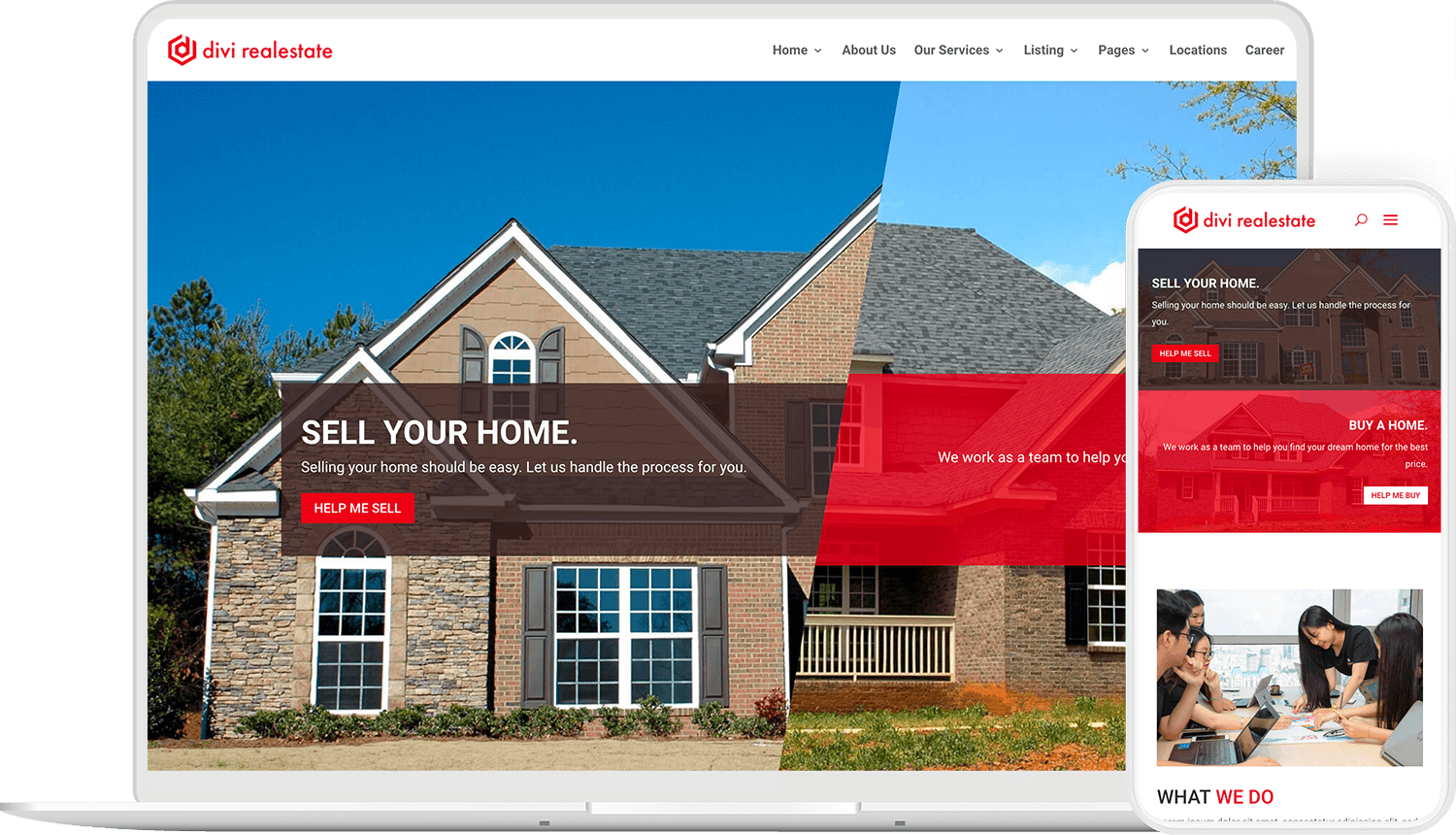This landscape-oriented photo features a detailed screenshot of a company's website displayed on what appears to be an iPad with a thin white border. The device has a rectangular shape with rounded edges and is framed in a grayish color. The top section of the website includes a white navigation bar with red text bearing the company’s name, "Divi Real Estate," written as D-I-V-I alongside a red icon featuring a 'D' with an open-top right border. 

Toward the right of the navigation bar, menu options are displayed sequentially: Home, About Us, Our Services, Listing, Pages, Locations, and Career. Below the navigation bar, there's a large image of a house set against a backdrop of a blue sky and trees, overlaid with a transparent gray box. This box contains the text: "Sell Your Home. Selling your home should be easy. Let us handle the process for you." Beneath this, a red button reads "Help Me Sell."

Further down, the website showcases a photo of the same app displayed on a phone, which is similarly framed by a white border. The app's interface shows vertically stacked options, including "Sell Your Home" and a red text box that says "Buy a Home." There is also an image featuring a group of people sitting around a desk, suggesting a collaborative environment.